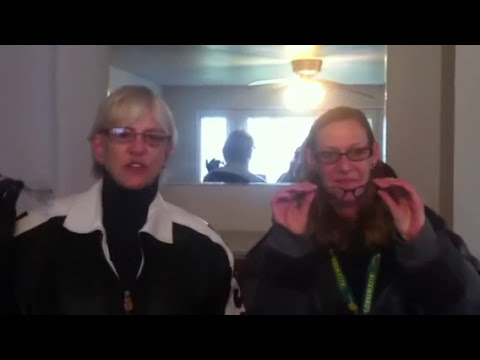This photograph captures two women in a warmly lit room, perhaps a living room, with a large mirror on the wall behind them that reflects the back of their heads and a ceiling light. On the left, the blonde-haired woman, who appears to be mid-sentence, wears black glasses with a white-collared black jacket over a black turtleneck. The woman on the right, who has long dark brown hair and black glasses with thicker frames, also holds another pair of glasses with thinner frames in her hands. She is adorned in a dark jacket with a green lanyard around her neck and has a subtle smile on her face. The golden glow from the ceiling light adds a warm ambiance to the scene.